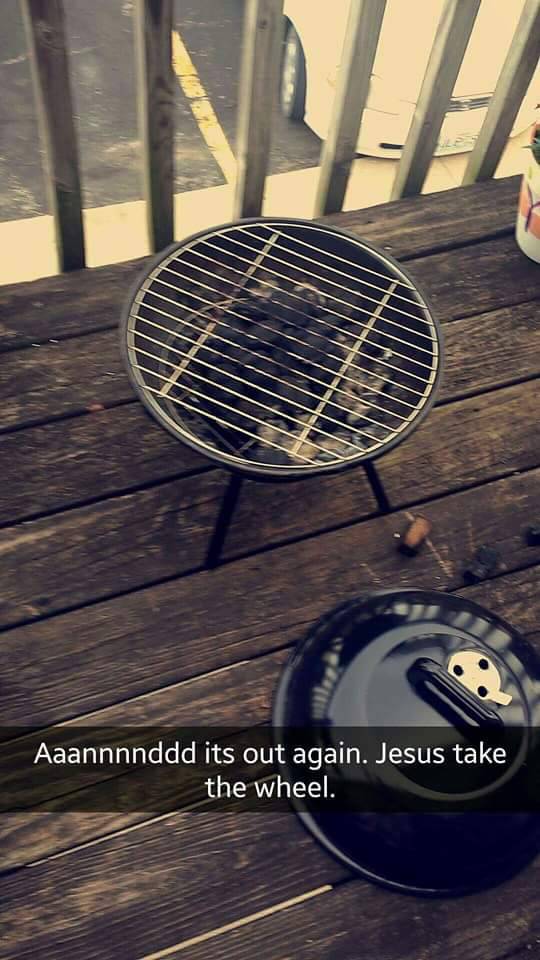The photograph captures a detailed top-down view of a small, squat, three-legged charcoal grill situated on a raised wooden deck or patio. The deck is constructed from dark brown wood that extends horizontally from left to right and features a wooden railing with several vertical spindles at the top of the image. The grill itself is centrally positioned, though slightly towards the top, with its black metal lid placed off to the side towards the bottom of the picture. Inside the grill, there is a metal slotted plate above blackened, burnt chunks of charcoal. In the upper background, partially visible, is a parking lot with a parked car, while the lid of the grill, resting on the ground, adds to the sense of an outdoor cooking scene. The semi-transparent black banner across the image, with white text, reads "and it's out again Jesus take the wheel," punctuated dramatically and humorously with "A-A-A-N-N-N-N-D-D-D" repeating the word 'and.' The color palette includes off-whites, various shades of black, gray, and dark brown, enhancing the rustic and somewhat whimsical atmosphere of the scene.